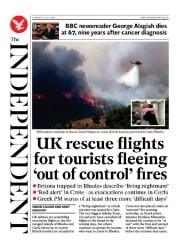This image depicts a news page from a British newspaper. In the top left corner, there is a red circle with a blurry logo inside, which appears to be a bird, possibly an eagle. Along the left side of the page, the text "INDEPENDENT" runs vertically in large, bold type. The headline states, "BBC news reader George [blurry text] dies at 67, nine years after cancer diagnosis." To the left of this headline is a photograph of a man.

Beneath this, there is a large, striking photo of a forest engulfed in flames. The sky is filled with heavy clouds of smoke, and a helicopter can be seen flying off to the right. In the bottom right corner of this forest scene is an inset image showing two people hugging each other inside a building. The caption for this inset image is too blurry to read.

The main headline reads, "UK rescue flights for tourists fleeing out-of-control fires." The following text is partially legible and mentions people "trapped in roads describe living a nightmare." Below this text, a red dot precedes the words "red alert in [blurry text], as evacuations continue in [blurry text]." Another red dot highlights a warning from the Greek Prime Minister about at least "three more difficult days" to come. The article below this headline contains blurry, unreadable text.